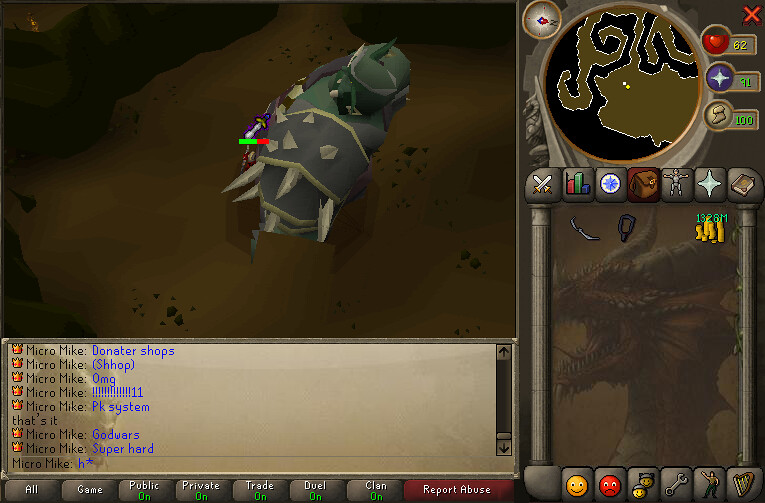This image is a detailed screenshot from the video game RuneScape. Dominating the top left two-thirds of the image is an overhead view of a green-skinned, orc-like character clad in silver armor adorned with white spikes. The most prominent of these spikes are on the shoulder plate, which has several smaller spikes on top and longer ones protruding from the side. In front of the character is a circular health meter showing two-thirds green and one-third red, indicative of the character's remaining hit points. Below this action scene, the chat box is busy with the player's dialogue. A character named Micromikes is actively typing messages such as "Donator Shops," "SHOP," "OMG!!!11," "PK System," "God Wars," and "Super Hard," all of which are in blue text. 

The bottom of the screen features various buttons labeled "All," "Game," "Public On," "Private On," "Trade On," "Duel On," "Clan On," and "Report Abuse." To the right of the image, there is an overhead map with black and brown coloring to distinguish water and land, respectively. This map indicates where the player is located. Adjacent to this are three meters showing different statistics or resources, labeled 62 in yellow for health, 91 in green for prayer, and 100 in green for energy. Beneath these meters, there's a white prayer symbol set against a purple background and an icon of a running shoe. Finally, a piece of gold labeled "1328M" appears in the inventory screen at the bottom right, surrounded by various other icons.